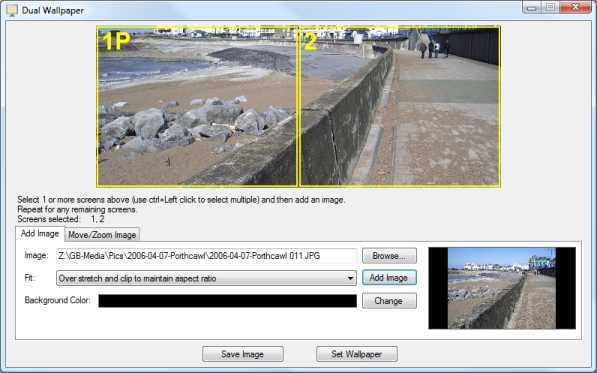The image is a rectangular, blue-bordered screenshot from a computer, showcasing a tool labeled "Dual Wallpaper" at the top. It features two vertically split sections of the same scene side by side. The left section is designated as "1P" and the right as "2," both marked in yellow text. The scene portrays a beach path with people walking, rocks in the foreground, and the ocean waves lapping close to the path, separated by a seawall.

Underneath the dual images, instructional text states, "Select one or more screens above (use Ctrl + left click to select multiple) and then add an image. Repeat for any remaining screens." The screen selection is shown as "1, 2." Further options include a grayed-out section with a "browse" button next to an "add image" button, as well as text boxes for "fit" options—offering choices such as "over stretch" and "clip to maintain aspect ratio." The background color option displays a black strip with a "change" button beside it.

To the right of these settings, a smaller thumbnail of the combined image appears, flanked by buttons labeled "Save Image" and "Set Wallpaper" at the bottom. Lastly, another section contains a gray "move/zoom image" tab alongside options to add images or adjust background and fit parameters, emphasizing the customization capabilities of the tool being used.